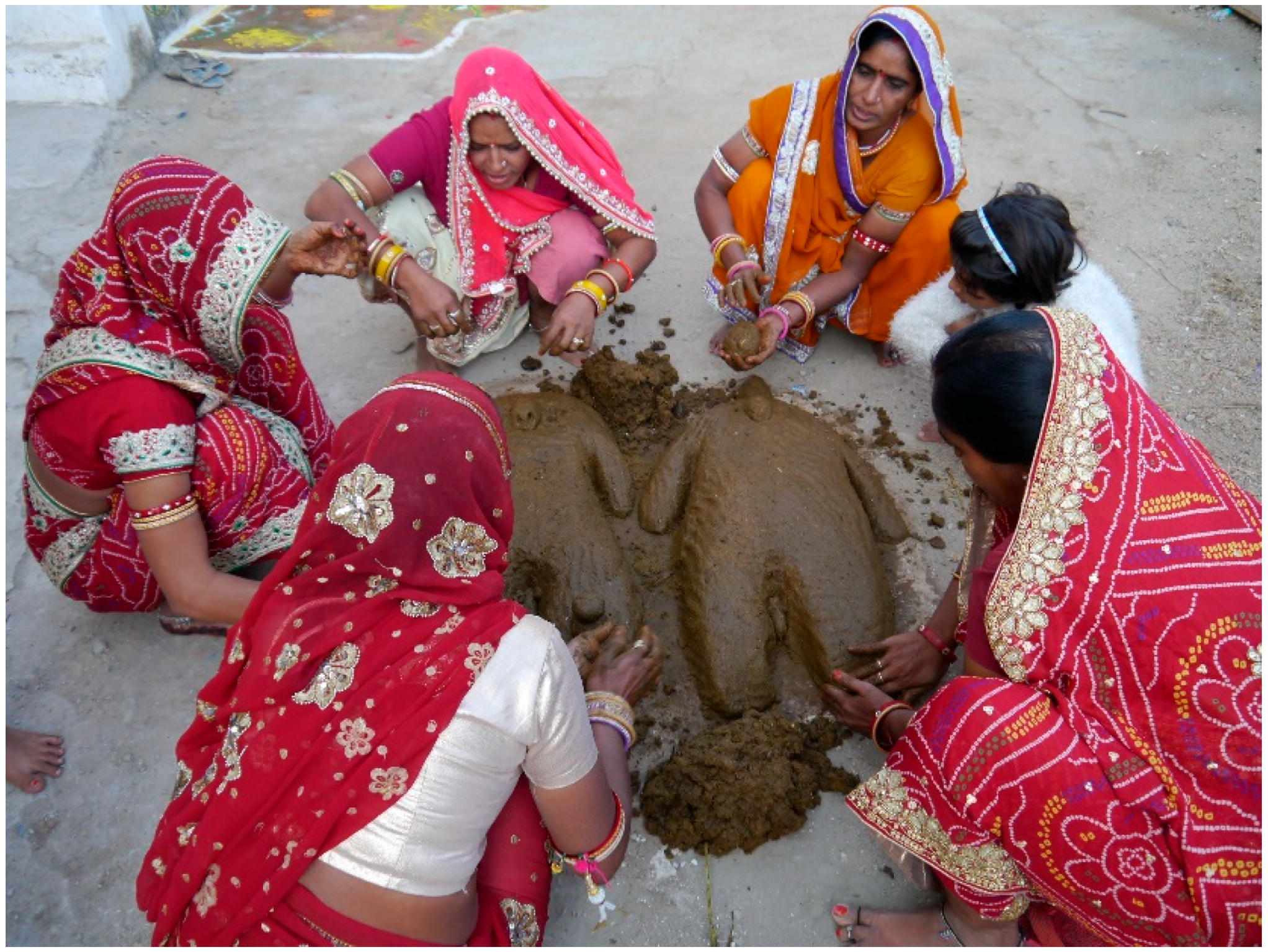In an aerial view of a typical Indian village courtyard with a cemented gray floor, six women are gathered in a tight circle, kneeling or squatting with their feet flat on the ground and leaning against their knees. They are deeply engrossed in sculpting human figures from bright brown mud or clay. Vibrantly dressed in traditional saris, the women are adorned with patterns and designs in shades of red, pink, and orange, some with gold and purple accents. Matching blouses, bangles, and other jewelry add to their colorful attire. Among them, a young girl stands out in a white dress with a white hair band. The communal scene is rich with cultural essence as the women artistically shape the mud on the concrete surface.